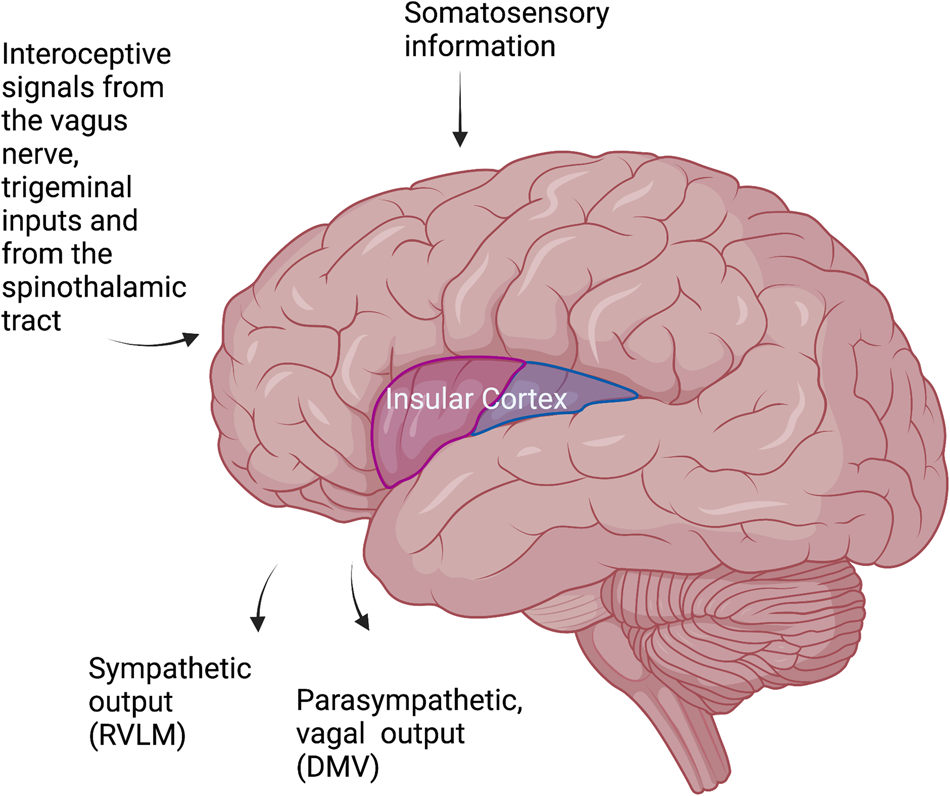This image features a simple illustration of a human brain viewed from the side, set against a white background. The brain is rendered in a light purplish-pink color. A specific region, the insular cortex, is distinctly highlighted in a reddish-blue color to stand out. The diagram includes various call-outs and arrows pointing to different parts of the brain, identifying the origins and destinations of multiple neural signals. Notably, it details interoceptive signals from the vagus nerve, trigeminal inputs, and inputs from the spinothalamic tract. Additionally, arrows illustrate somatosensory information and outputs, including sympathetic output (RVLM) and parasympathetic vagal output (DMV). The text conveying this information is in black, providing clear labels for each highlighted neural pathway and interaction within the brain's anatomy.